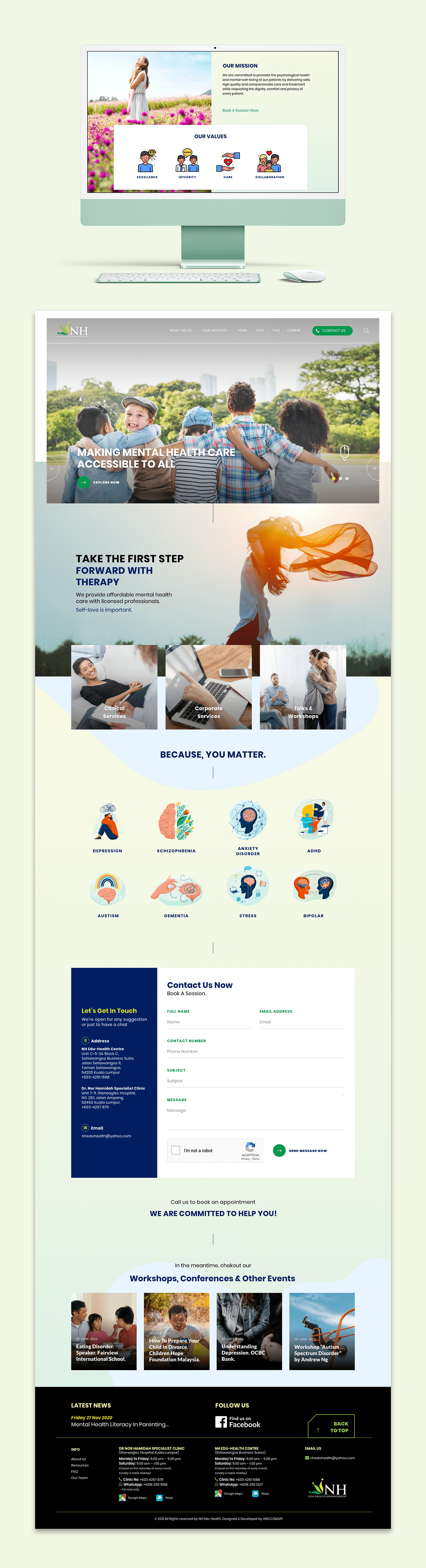The image appears to be a promotional display or a mock-up of a full web page for a mental health service. At the top, a narrow, light green box features a series of images. The first image in this box is of a narrow, elongated computer monitor with a greenish hue, displaying a screen with content similar to what is visible below. In front of the monitor, there is a keyboard and a mouse.

Below this section, there seems to be a detailed advertisement or the design layout for a complete web page. The headline is small and difficult to read, but it accompanies a wide, narrow picture showcasing a group of children playing. The prominent tagline in this section reads, "Making Mental Health Care Accessible to All."

Further down the page, there is another headline that declares, "Take the First Step Forward with Therapy." This section features an image of a woman running, with a scarf elegantly flowing behind her. Additional smaller pictures of various individuals are scattered throughout the layout, alongside some icons with text that is too small to decipher. The overall design indicates the web page is dedicated to offering mental health services.

In the lower right corner, there is a logo with the initials "NH," but the accompanying text is too indistinct to read.